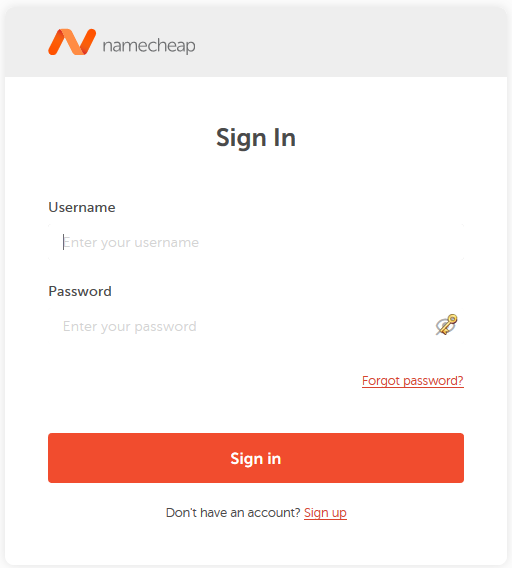The image features a split background, with the top portion in grey and the lower section in white. On the left side of the grey section, there is a stylized 'N' in a vibrant orange shade. To the right of the 'N', the text "Cheap Name" is displayed in a dark grey or nearly black color. 

The white section contains a login interface. Centrally positioned is the heading "Sign In" in bold black text. Below this, towards the left, the text "Username" is followed by a light grey input bar with a placeholder that reads "Enter Your Username." Below the username field, there is a password field labeled "Password." This field includes a toggle feature to show or hide the password. 

At the bottom of the login fields, there is a large orange button with the text "Sign In" in white, centered within the button. Below the button, centered in smaller text, it reads "Don't Have an Account?" with "Sign Up" underlined and in the same orange color as the 'N' and the button. The layout is clean and straightforward, aimed at facilitating easy access for users.